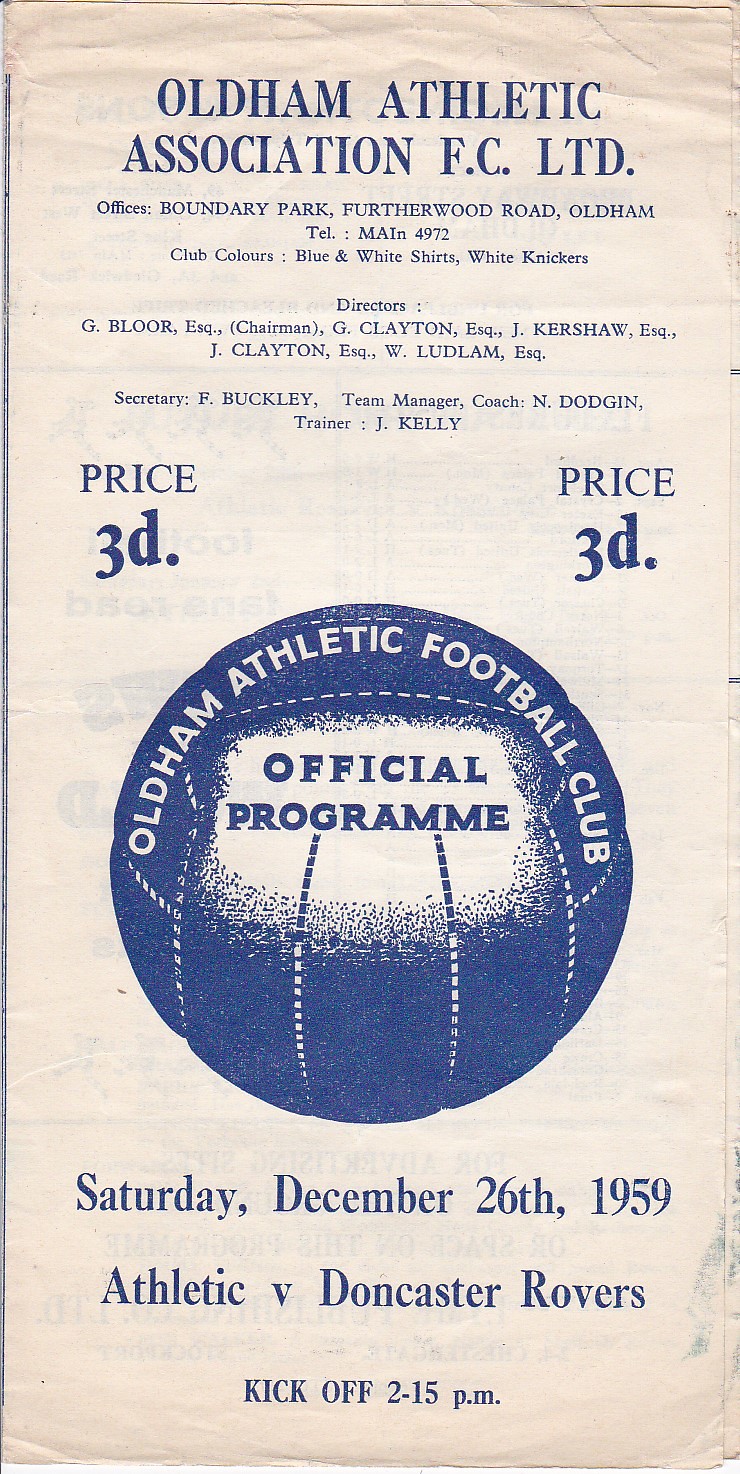The front page of this football club program, from December 26, 1959, features Oldham Athletic Association FC Limited prominently in dark blue letters across the top. The program, printed in dark blue ink on an off-white, slightly yellowed background, exudes a vintage aesthetic. Centrally positioned is a large, circular illustration of a soccer ball, encasing the white text "Oldham Athletic Football Club Official Program." Below this, details about the match are clearly stated: "Saturday, December 26, 1959, Athletic vs. Doncaster Rovers," with the kickoff time at 2:15 PM. The program is priced at 3d, implying an old currency denomination. The upper section also includes detailed information about club officials, such as directors, team managers, and other staff, framed within the blueprint style of the entire page.